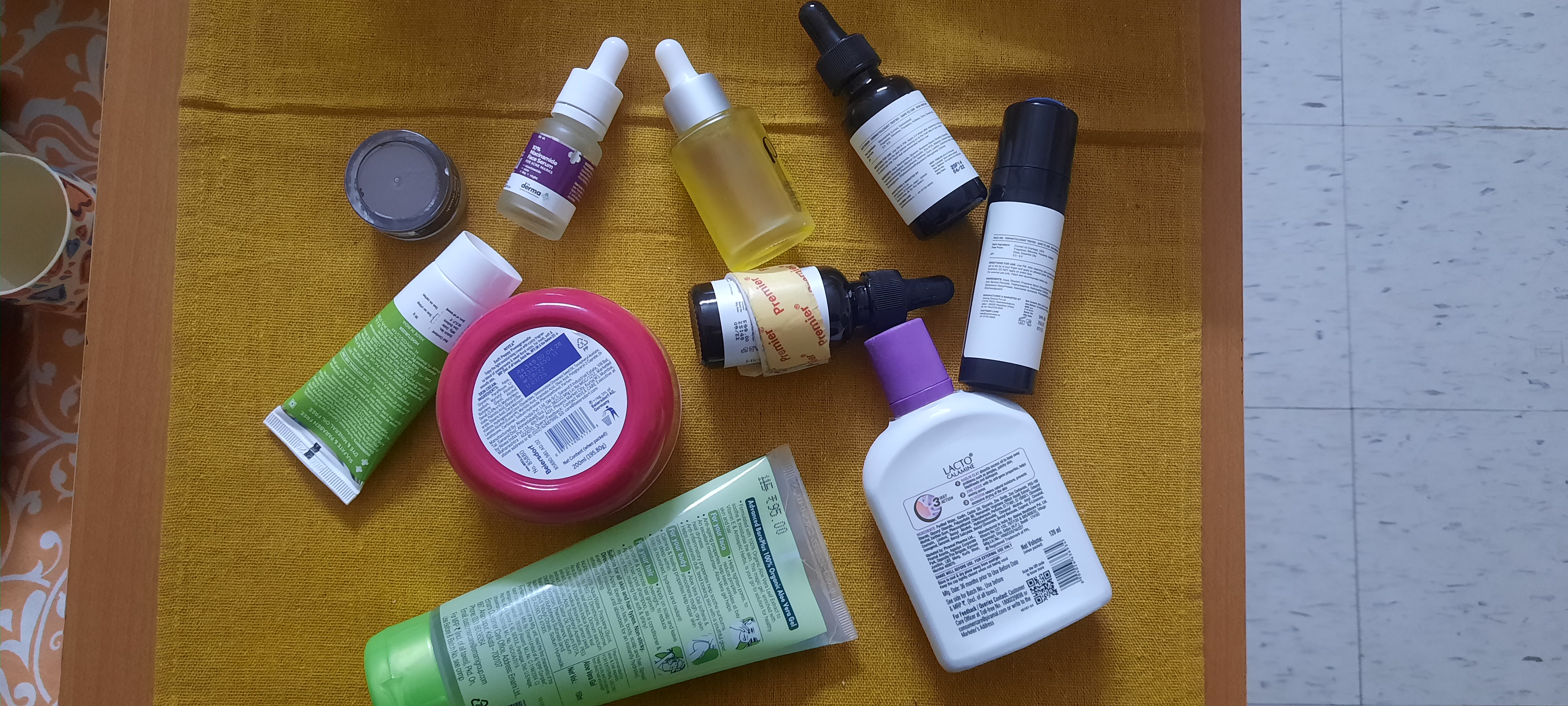A variety of skin care and beauty products are meticulously arranged on a yellowish cloth spread out on the ground. The products are strategically turned on their backside, hiding all brand names and logos. Among the assortment, there are serums in black containers with white labels, equipped with black droppers, and oils in clear bottles featuring white droppers. Additionally, the layout includes several tins likely containing lip gloss, and containers that suggest facial washes or scrubs. One notable circular container stands out with its distinct green body and red bottom.